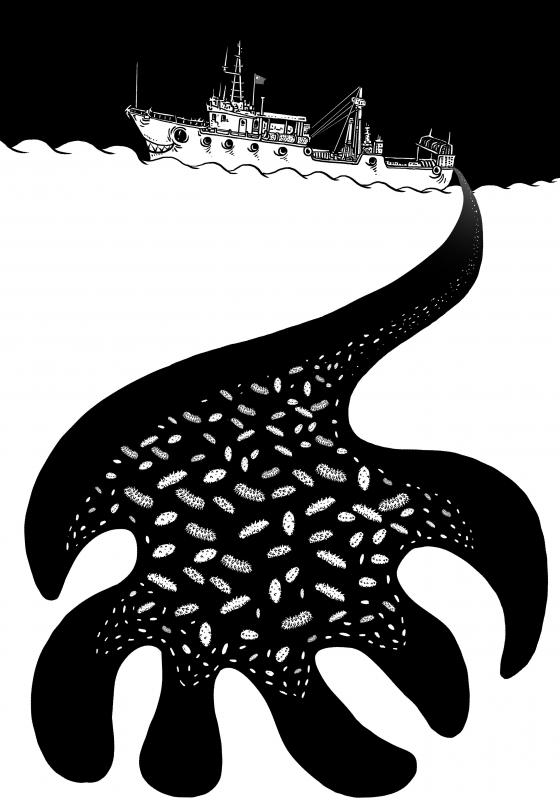This graphic depiction illustrates a fishing boat navigating an oceanic expanse. Crafted through computer-generated imagery, the scene adopts a stark black-and-white palette. The boat, characterized by its prow resembling a shark's face, floats over a white sea beneath a black sky. Trailing behind, a chaotic black spill invades the otherwise calm waters, dominated by six finger-like tentacles sprawling from its core. Within this dark mass, numerous tiny shapes, reminiscent of bacteria or amoebas, seem to writhe and float, suggesting a scene of pollution or the boat dispersing chum, further enhancing the eerie and unsettling atmosphere.